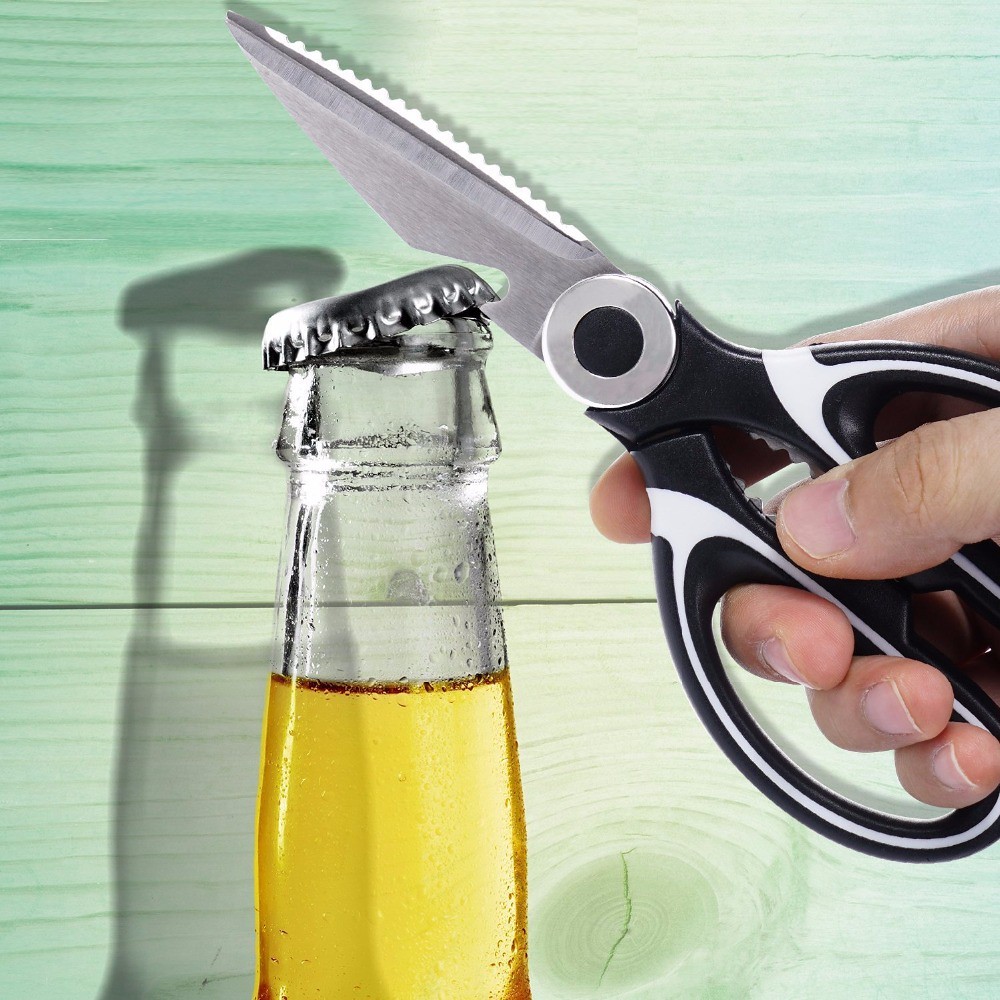The color photograph, set in a square orientation, showcases the intricate moment of opening a beer bottle in vivid detail. Positioned just left of center, the bottle's halfway-filled neck reveals a golden-yellow liquid, reminiscent of a Corona beer, capped with a silver top. A hand entering from the right manipulates a pair of black and white-handled metal scissors, utilizing the bottle opener feature on the bottom blade to pry the cap loose. The scissors notably have a jagged-edged blade. Behind the bottle, wooden paneling with a lime greenish tint serves as the backdrop, displaying distinct wood grains and a knot in the lower right corner. The light casts a perfect silhouette of the bottle against the green-stained wood, adding depth and interest to the scene.